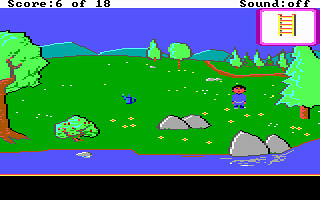Screenshot of an old-school, 8-bit video game featuring a serene, grassy landscape dotted with seven trees and a shrub. The top left corner displays the score as "6 of 18". A river flows diagonally from the bottom right to the bottom left of the image, bordered by a few grey rocks. The sky is clear and blue, casting an idyllic aura over the scene. A dirt road starts at the middle right and extends towards the central horizon, inviting exploration.